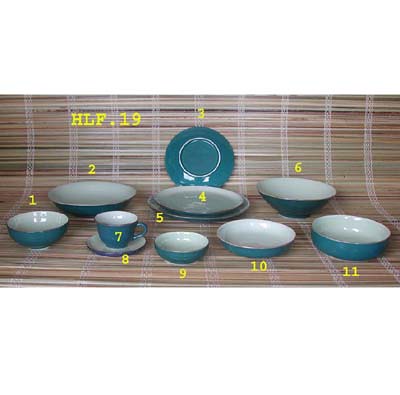The image depicts a coordinated set of dinnerware consisting of 11 items arranged on what appears to be a bamboo-style mat with visible stitching lines. The dinnerware set includes various plates, bowls, a saucer, a cup, and two circular pans. All items share a white inner surface and a tealish blue outer surface, giving them a fresh, clean, and enamel-like appearance. 

The set is methodically organized and numbered: 
1. A smaller bowl on the left.
2. A larger bowl positioned behind it.
3. A plate standing upright to display its teal blue bottom.
4. An identical plate laid flat beneath the upright one.
5. A larger plate situated under the flat one.
6. A medium-sized, taller bowl.
7. & 8. A teacup and saucer set to the front left.
9. A small bowl in the front.
10. A smaller circular pan.
11. A larger circular pan.

The arrangement also features yellow text in the top left corner that reads "HLF.19," presumably to label or categorize this dishware collection.